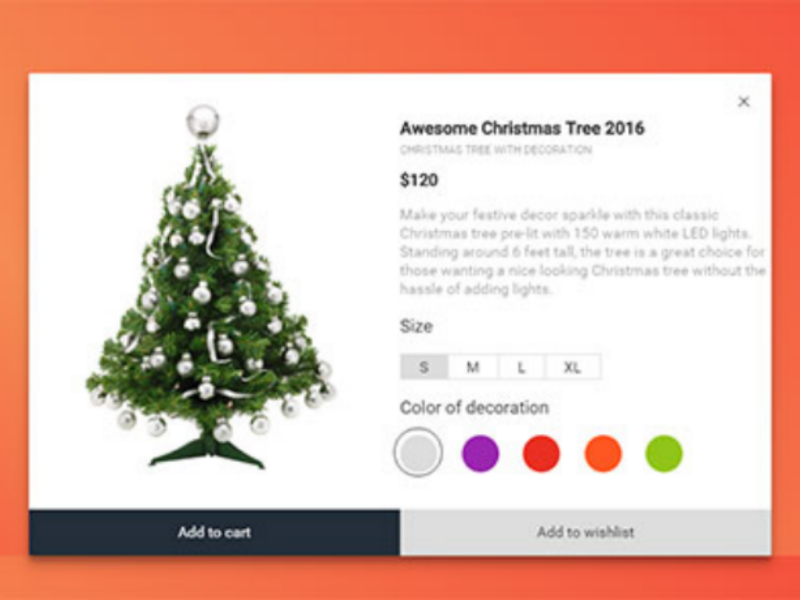A blurry image captures someone in the act of either ordering or browsing for Christmas trees online, though the specific website remains unclear. The background features a gradient of orange hues, transitioning from a normal orange in the top left to a reddish-orange in the top right, with lighter shades of orange at the bottom left corner. The foreground is dominated by a window with a white background.

Occupying the left half of the picture is a plastic green Christmas tree adorned with dark green tripod feet. The tree itself is dark green and decorated with silver ornaments, including variously sized silver balls and silver tinsel. A large silver ball sits atop the tree, while smaller silver balls are scattered throughout its branches.

Below this image, a dark blue button offers the option to "Add to Cart," and towards the bottom right of the screen, a grey button allows users to "Add to Wishlist." There are options to select the color of the ornaments, with choices including grey, purple, red, orange, and light green, although the tree will remain green. Additionally, users can choose the size of the tree, which is referred to as the "2016 Christmas Tree" and priced at $120. The available sizes are small, medium, large, and extra-large, with the small size currently selected.